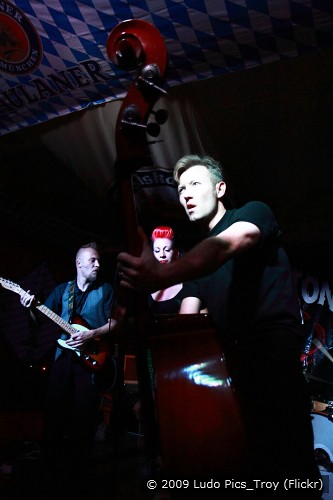In this portrait-oriented photograph, three Caucasian musicians perform on a dimly lit stage. The spotlight focuses predominantly on the man closest to the camera, a blonde guitarist. His hair is buzzed on the sides but longer on top, and he is dressed entirely in black. His mouth is slightly open as he looks out towards the crowd, engaging directly with the camera lens. 

Centrally positioned behind him, a woman with striking, fire-engine-red hair peeks out, her hair cut short. She wears a black sleeveless top, and while her instrument isn't clearly visible, she plays a significant role in the ensemble. 

To the right, another man plays an instrument that resembles a cello, indicated by the long neck visible at the top of the picture. This man, sporting a short buzz cut, dons a blue vest over a black t-shirt. He looks towards the woman with the red hair, creating an interactive dynamic between the band members. 

The scene is set in darkness, with the spotlight providing the critical illumination that defines the subjects and their instruments. Above them, the ceiling displays a piece of cloth or paper adorned with blue and white checks, adding a unique backdrop to the otherwise dark stage. In the bottom right corner, a watermark reads "© 2009 Ludopix_Troy (Flickr)," indicating the photograph's copyright.